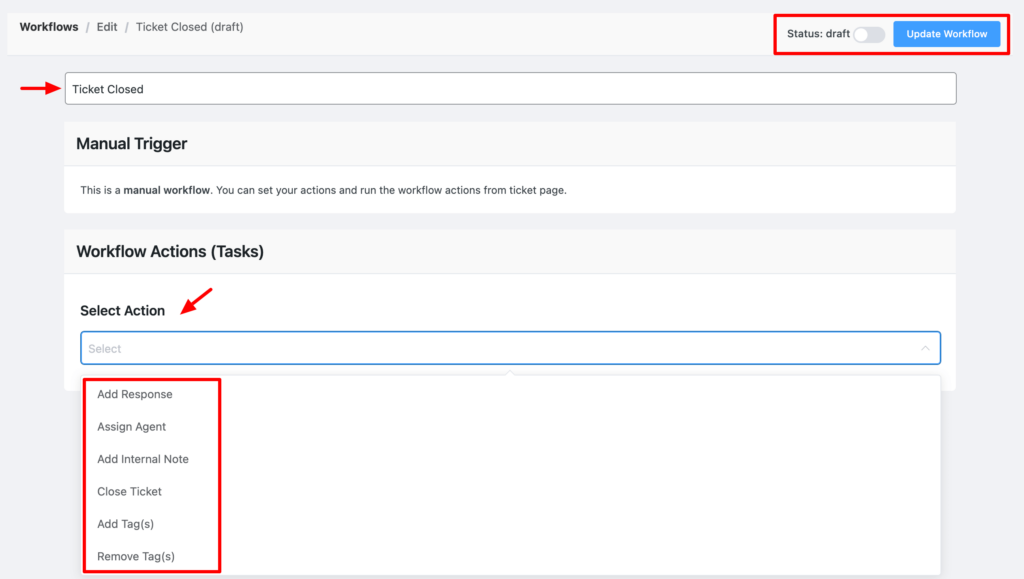The image depicts the "Workflows / Edit / Ticket (Draft)" interface with various elements marked for emphasis. At the top left, the title reads "Workflows / Edit / Ticket (Draft)," while the top right corner indicates the status as "Draft." A toggle bar, currently in the off position, is visible.

Highlighted with a red box is a prominent blue button labeled "Update Workflow." Below this, another red arrow points to a text box containing the label "Ticket Closed." Further down, there is a section titled "Manual Trigger," denoting that "This is a manual workflow. You can set your action and run the workflow action from the ticket page."

Beneath this, a heading reads "Workflow Actions" followed by "Task (Select Action)," which is also pointed out by a red arrow. An empty text box is positioned below this heading, with another red box drawn around the words located to the left of this text box, underscoring them.